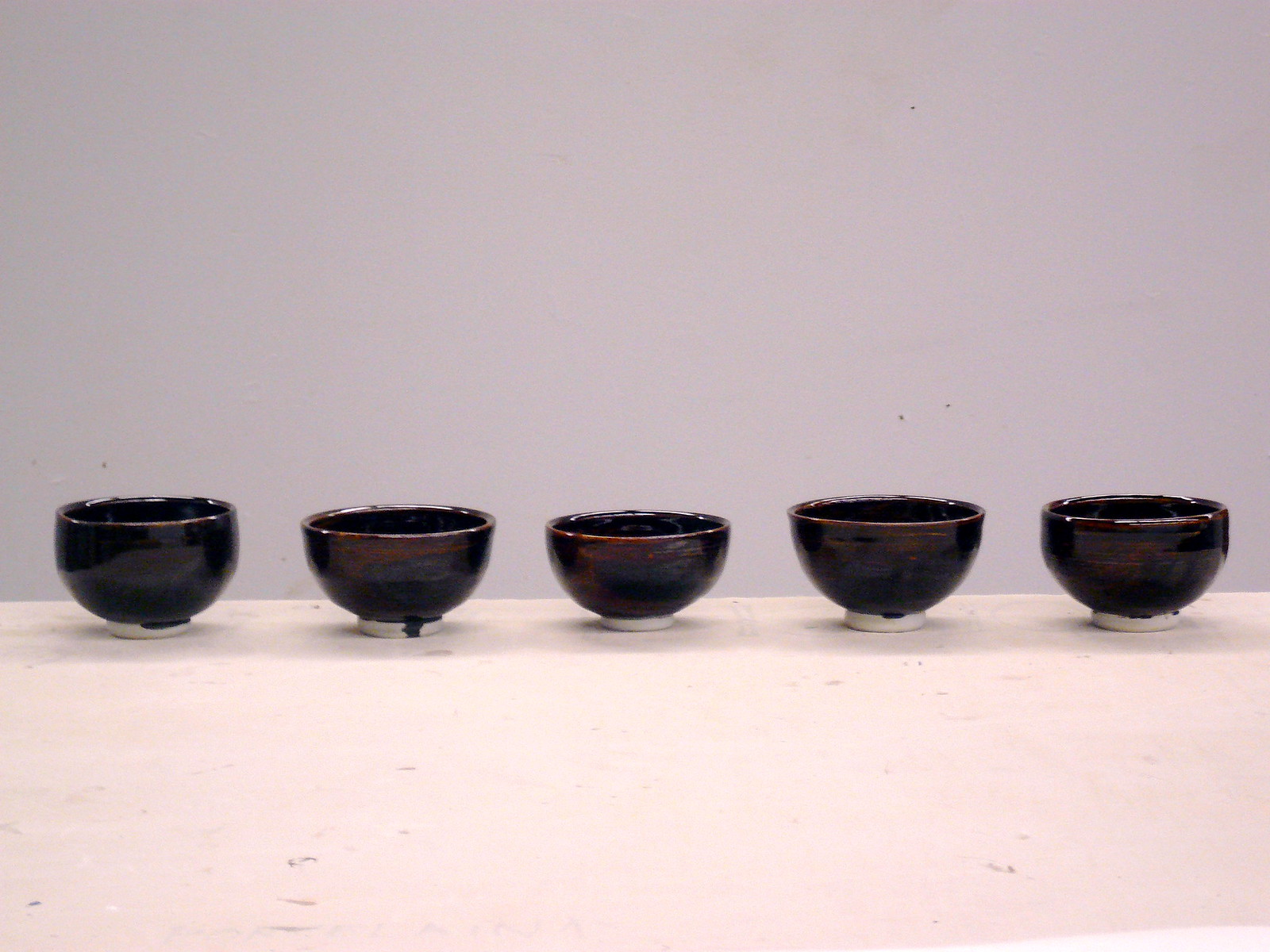The photograph features five handmade ceramic bowls, arranged in a line on a white surface that extends beyond the frame, possibly a long table ending against a white wall. The backdrop is a reflective whitish-gray, illuminated slightly by a flash. Each bowl showcases a dark glaze with a deep brown-red tinge, creating an artistic and cohesive design marked by unique variations. The glaze doesn't reach the bottom, leaving the base an unpainted beige, revealing the natural clay. The bowls differ slightly in size, suitable for large salads or as display pieces in a living area or kitchen. Notably, the glaze has dripped in some areas, adding character to each piece—particularly the second bowl from the left, which has a prominent drip on its base. This collection embodies a handcrafted aesthetic, ideal for a centerpiece or conversation starter.